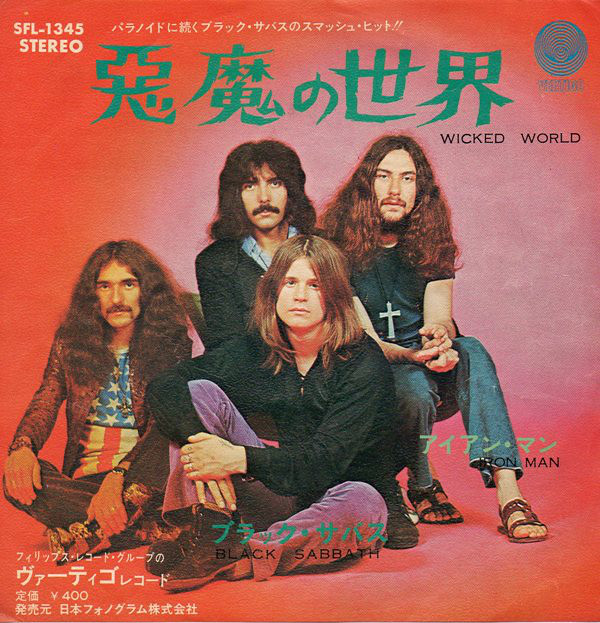The image is of a vintage Japanese vinyl album cover of the iconic rock band Black Sabbath. The cover features the four members, including Ozzy Osbourne at the forefront, all dressed in white and gazing ahead. They are seated against a red backdrop, with three of the members sporting mustaches and shoulder-length hair. Prominent green Japanese text adorns the upper center, translating to Wicked World, Iron Man, and Black Sabbath in black lettering below. Additional Japanese text is scattered around the lower center, right, and left of the cover. The top left corner features the text "SFL-1345 Stereo," while a blue logo sits in the upper right. The upper corner also includes more Japanese lettering, suggestive of the album’s international edition. Overall, it captures the classic and influential essence of Black Sabbath, visually appealing to both vintage vinyl collectors and fans of the band.